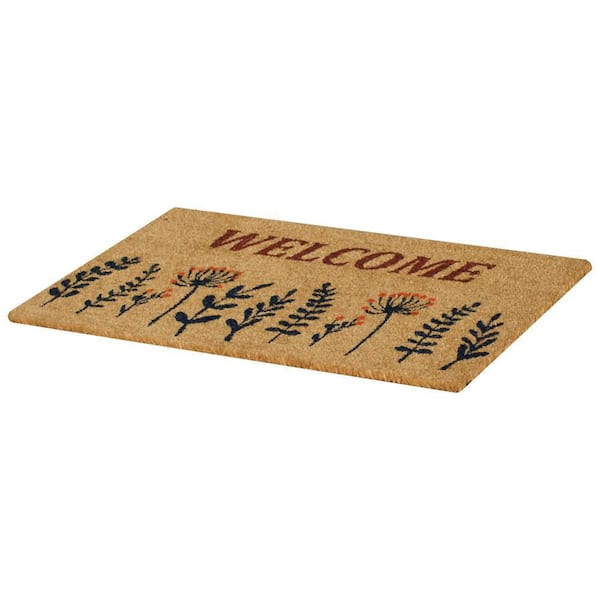This image showcases a rectangular welcome mat placed on a white background, viewed from the ground level on the right side. The mat is a light brown or tan color, composed of a firm, textured material resembling rubber or nylon, designed for effectively cleaning dirt off shoes. The word "WELCOME" is prominently displayed in all capital letters with a reddish-brown or burgundy font at the top part of the mat. Below this text, the bottom half of the mat is adorned with an array of botanical designs. These include curvy vines and fern-like elements with small circular teardrop-shaped leaves and stems. Among these, there are individual branches of eucalyptus-like leaves and flowers with small orange buds at the tips. The intricate botanical patterns are primarily green but include touches of orange and red, adding a natural, inviting aesthetic to the mat.